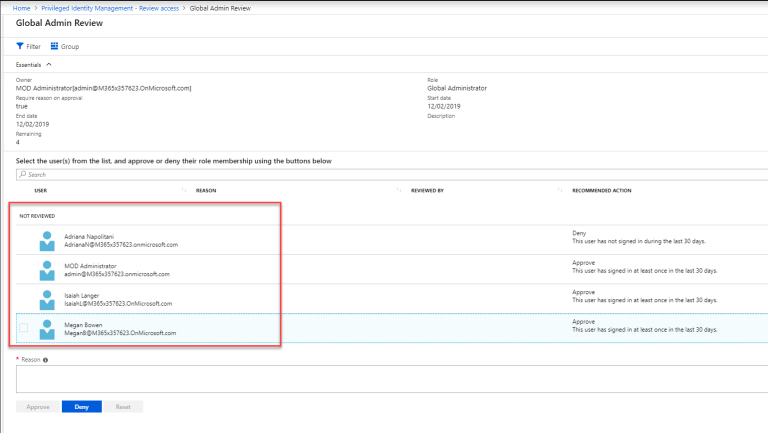**Detailed Caption:**

The image showcases a webpage dedicated to a global admin review process. At the top of the page, there are several navigation options, including "Home," "Privilege Identity Management," "Review Access," and the current section, "Global Admin Review." Just below these options is a filter feature and a "Group Essentials" section that displays key details such as owner information.

The "Group Essentials" section reveals the owner as an MOD administrator with the email "admin@M365Microsoft.com." It specifies that requiring a reason for approving actions is set to "true." The role in question is a "Global Administrator," with both the start date and end date listed as 12-02-2019. There are four remaining actions needing attention.

Further down, instructions guide the user to select individuals from a list and either approve or deny their role membership using the provided buttons. The table below these instructions includes columns for User, Reason, Reviewed By, and Recommended Action.

Users listed include:
- Ariana (last name not specified), recommended action: deny, with the reason being that this user has not signed in during the last 30 days.
- MOD Administrator, recommended action: approve, as this user has signed in at least once in the last 30 days.
- Isaiah Langer, recommended action: approve, also due to signing in at least once in the last 30 days.
- Megan (or possibly Bowen), recommended action: approve, again for signing in at least once in the last 30 days.

At the bottom of the page, there is a field for entering a reason and options to approve, deny, or reset actions.